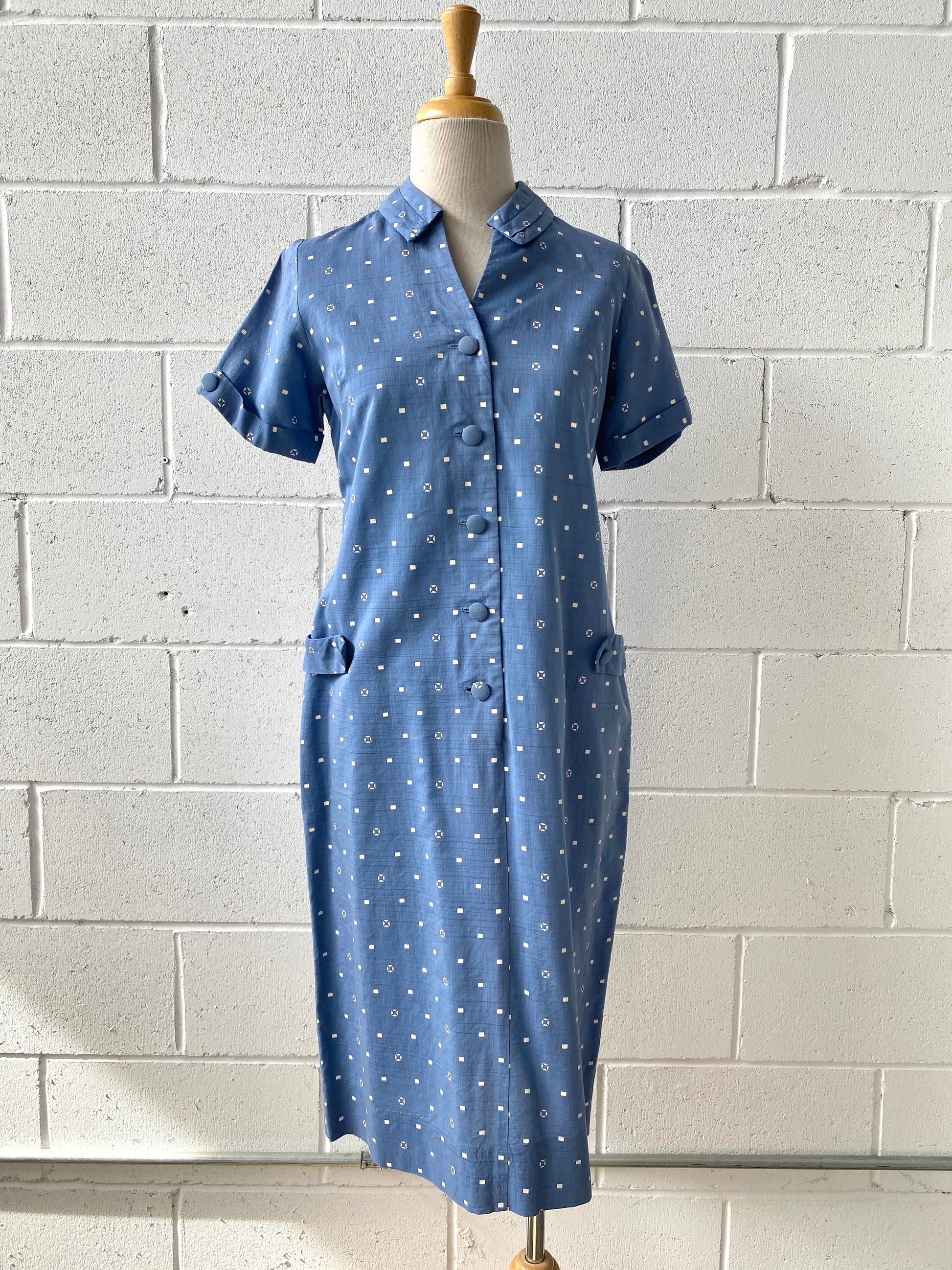This is a highly detailed photograph taken indoors during the daytime, capturing a mannequin positioned against a grey or white painted concrete block wall. Sunlight illuminates the wall, emphasizing the setting. The mannequin, headless and legless, features a white body with a wooden knob on top and a wooden base at the bottom, supported by a metal pole.

The mannequin displays a long, ankle-length blue dress adorned with white polka dots and other circular designs with blue centers. The dress is characterized by short sleeves with upturned edges, a collar, and a V-shaped opening where five buttons align down the front. There are two pockets on either side of the hips. The dress and its details are rendered crisply against the plain, textured background.